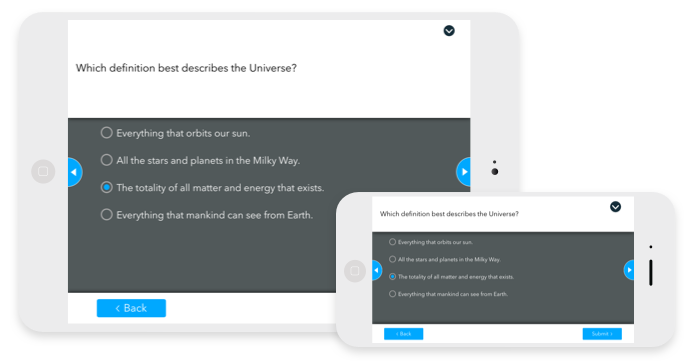Screenshot of a Computer-Generated Quiz Page

The image features a computer-generated screenshot of a quiz page. The visual, with a flat, two-dimensional aesthetic, portrays an iPad and a mobile phone positioned side by side. Both devices are rendered in a grayish-white color, each equipped with an on-off button. 

The focus of the quiz appears on both devices' screens, showing the same content. A white bar with a drop-down menu crowns the top of the quiz page. Below this, a black border separates the question and the multiple-choice answers. The question reads: "Which definition best describes the universe?" 

The multiple-choice options provided are:

1. Everything that orbits the sun
2. All the stars and planets in the Milky Way
3. The totality of all matters and energy that exists (selected)
4. Everything that mankind can see from Earth

Below the answer choices, navigation buttons are visible, featuring a 'Back' button in blue and a 'Next' button with arrow icons pointing left and right.

The overall design is minimalistic and lacks any additional text or intricate detail.